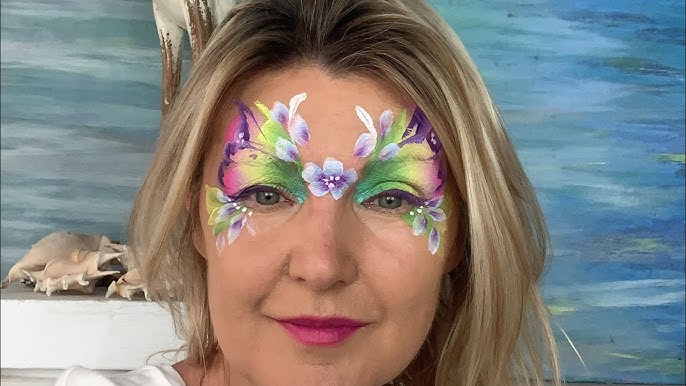The image depicts a close-up view of a woman with highlighted blonde hair, possibly in her 50s, wearing pink lipstick and a white shirt that is partially visible. Her face is adorned with intricate face paint featuring multi-colored floral designs, with green, yellow, pink, and purple hues, and dotted details along the lash line. Central to her forehead, between her eyes, is a prominent blue flower with a purple center. Her eyeshadow extends over her eyebrows, creating a cohesive painted look. She is seated or standing in front of a background featuring blue horizontal streaks and a ledge with seashells, adding to the image's aesthetic. The photograph is slightly blurry and crops out her chin and the top of her head, focusing on the detailed facial artwork that resembles butterfly wings. The woman wears a slight smile, contributing to the whimsical and artistic quality of the image.